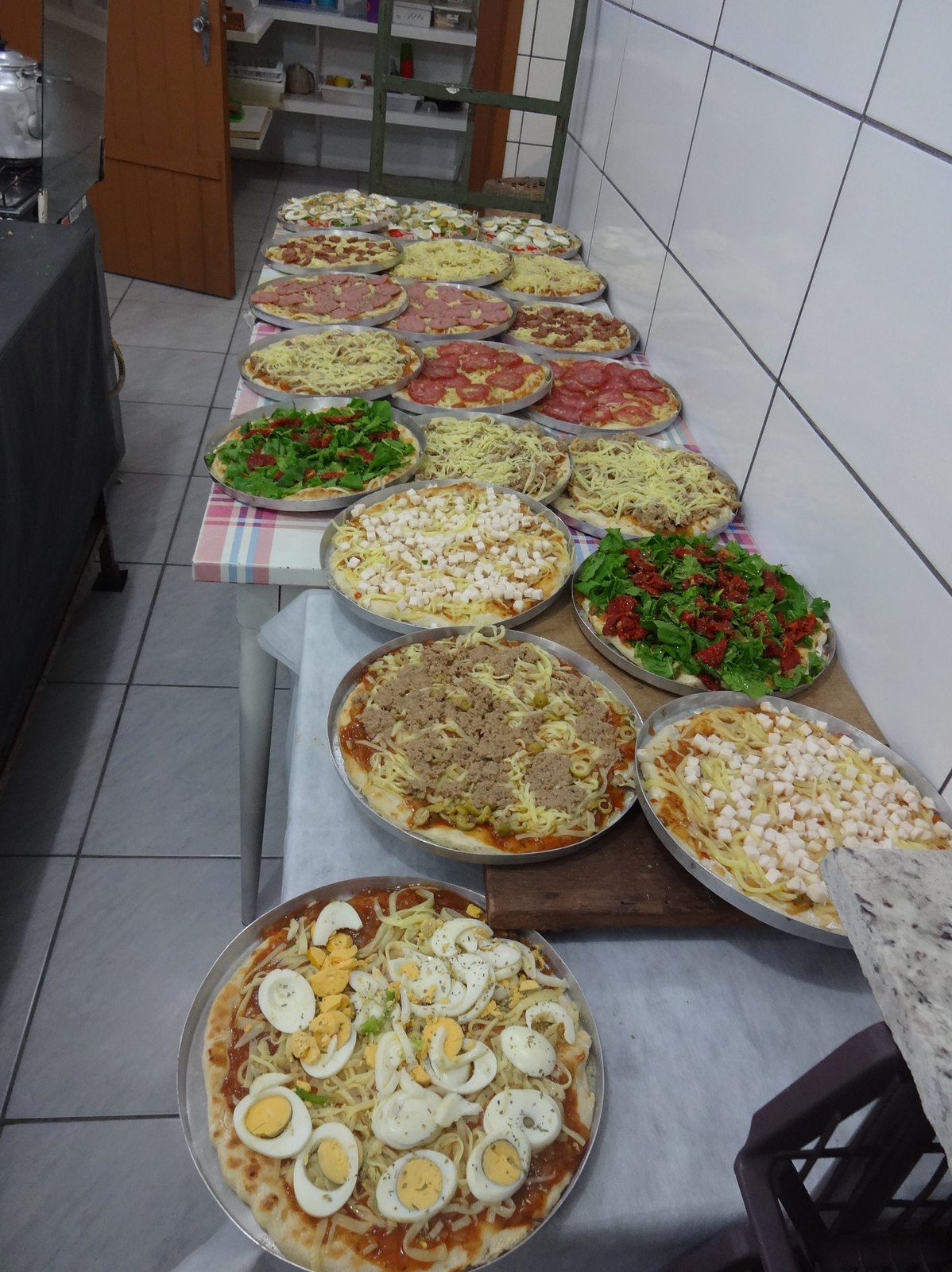The image depicts an indoor setting with large, shiny white tiles on the walls emulating a clean, bright atmosphere. The floor is covered with muted gray tiles that complement the sophisticated look of the space. Along the right wall, there are several tables adorned with different colored tablecloths: one table is covered with a black tablecloth, another with a light blue tablecloth, and a third donning a white, pink, and blue plaid tablecloth. These tables are laden with 20 trays of unbaked pizzas, each one carefully prepared with a variety of toppings. The toppings include items like eggs, meat, marshmallows, greens, and even pasta, adding a whimsical variety to the potential flavors. In addition to these tables, there is also a wooden cutting board present. A wooden door at the back leads to a closet with shelves inside. Another part of the room hosts a mechanical device, possibly an oven or a storage unit, enhancing the utility of the space. The overall impression is that of a well-organized room, perfectly set up for a pizza party with a diverse array of ingredients ready to be cooked.